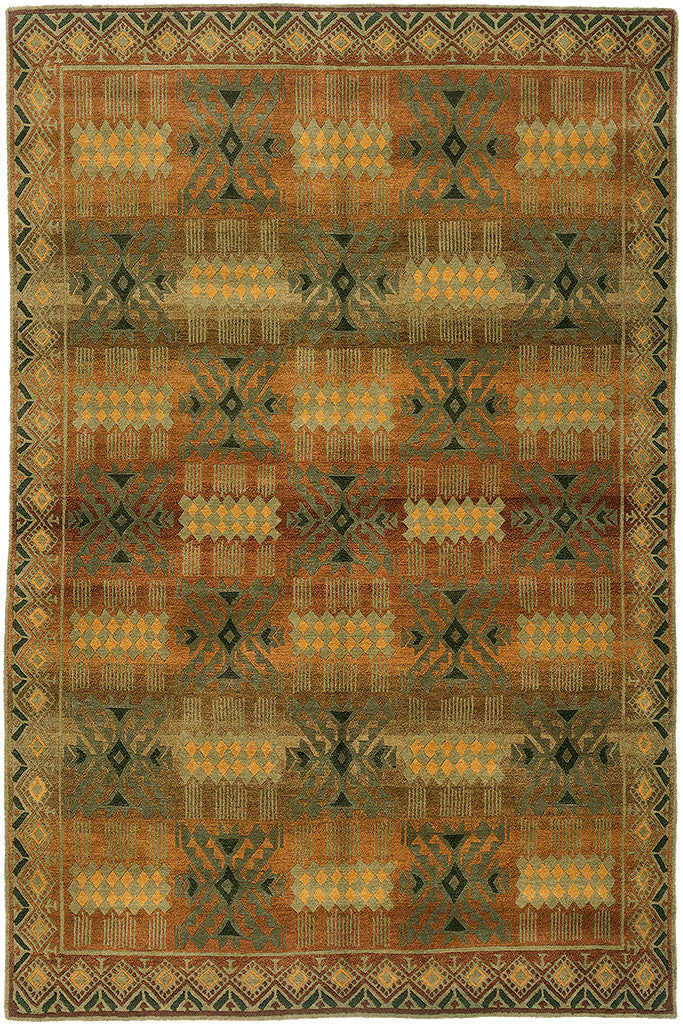The image depicts an exquisite, vertically oriented rectangular rug or tapestry, displaying a rich and intricate design. The rug is adorned with beautifully woven patterns and a muted color palette that includes gold, tan, black, greens, very light orange, and potentially darker shades of brown. The central tapestry features an overlay of bars of very light green with little orange flame-like designs. Various patterns dominate the rug, including repeating diamonds of orange and gold, surrounded by chevrons in a sawtooth style, and scattered black chevrons and arrows. The edges are decorated with a zigzag or chevron pattern of rhombuses and other geometric shapes, including squares that appear disconnected yet harmoniously placed. The entire rug's design is brought to life through the precise interplay of earth tones and geometric intricacies, making it not only visually striking but also suggesting an artisan’s painstaking craftsmanship. The setting is well-lit, ensuring the clarity and prominence of the rug’s details.